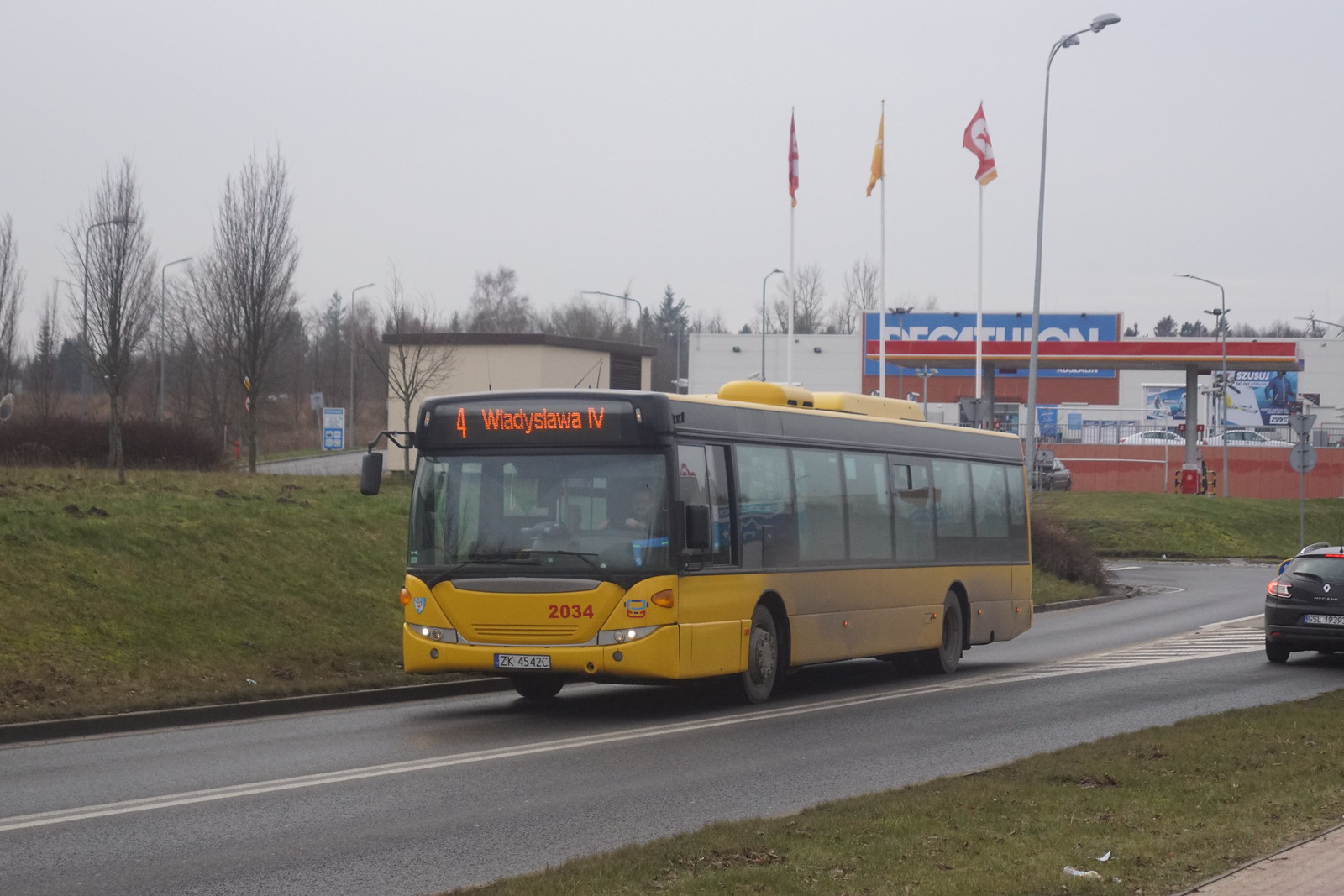This detailed daytime photograph captures a modern yellow and black transit bus rounding a corner onto a two-lane road, with its destination marked as "Wattishawa" in orange on the top bar. The bus, which sports tinted large windows and the numbers 2034 on its grill, appears to be a city bus rather than a school bus, indicating it's a tour or city transit vehicle. The scene is set on an overcast, gray day in what seems to be winter, given the bare trees and brownish grass in the median and roadside banks. 

In the background, there is a gas station with a distinctive red awning and a company store's name displayed in blue and white letters. Three flagpoles with flags and a tall light post stand near the gas station. To the right of the bus, a black SUV is heading towards the gas station, having just hit its brakes. The overall atmosphere of the photo is dreary, with no sunlight and no pedestrians, emphasizing the bus and vehicle movement in this urban setting.